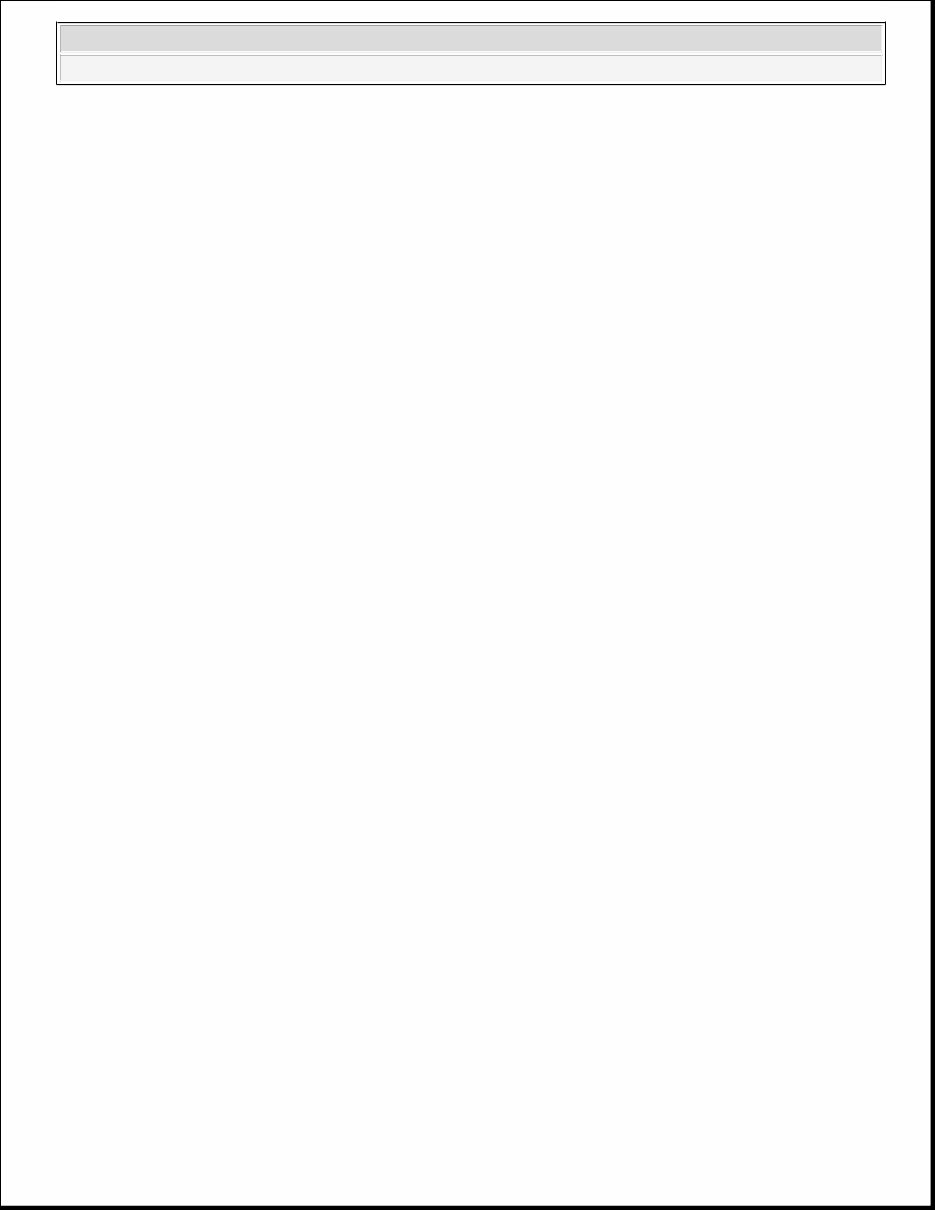This image features a predominantly black background with a distinctive element at the top. There is a very thinly-bordered black rectangle spanning nearly the entire width of the image. Inside this rectangle, two horizontal gray bars are present: the top bar is a darker shade of gray than the one below it. These bars occupy a minimal vertical space but stretch from one side of the image to the other.

The entire rectangle is outlined with a narrow black line on the top and left sides, while the right and bottom sides are bordered with a noticeably thicker black line. The rest of the image is entirely blank and devoid of any additional elements, giving it an unfinished or minimalistic appearance.

Overall, the design might represent the early stage of a webpage layout, potentially hinting at the beginnings of a menu bar at the top with the gray lines, against a blank canvas awaiting further development.